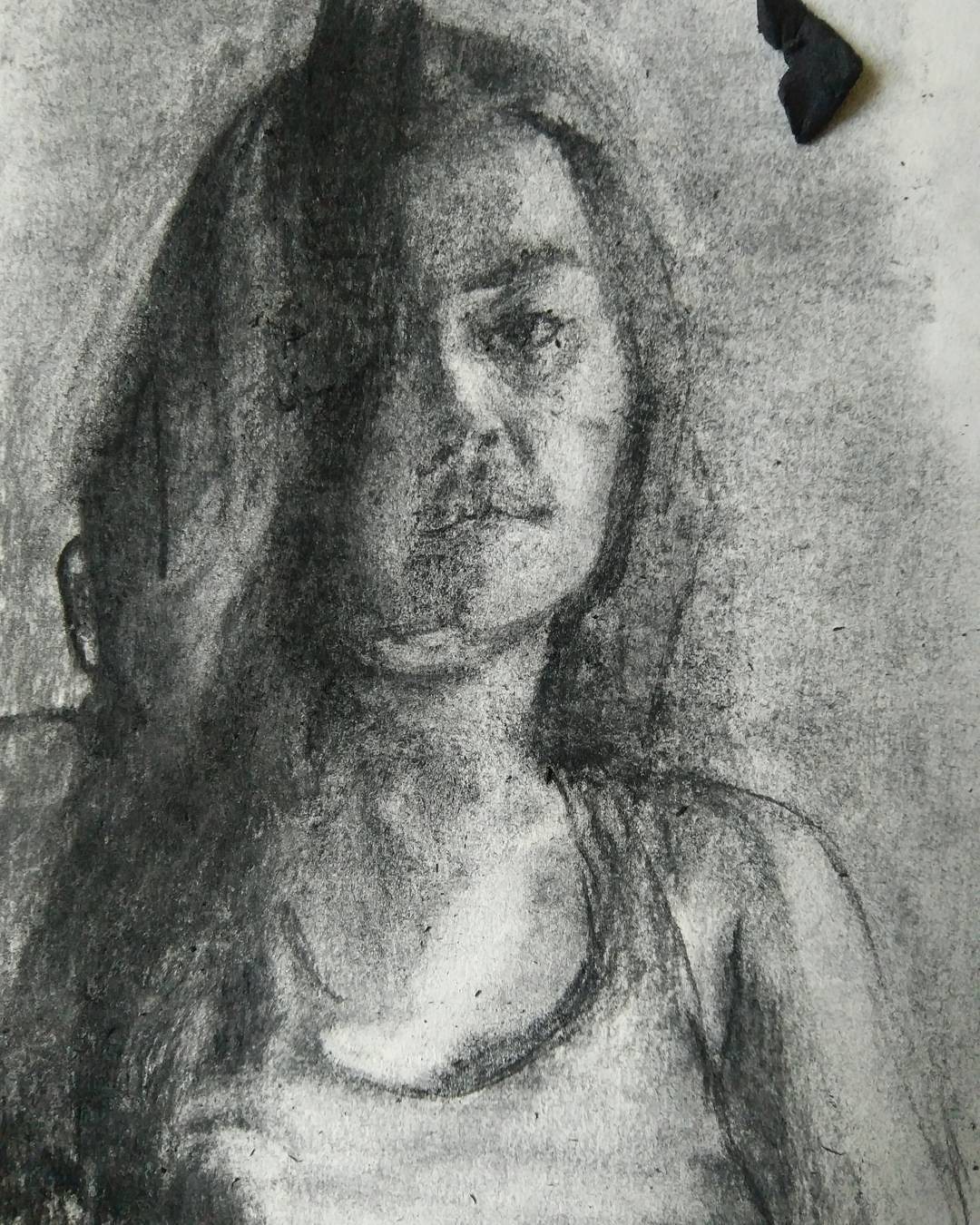This charcoal drawing portrays a young woman gazing directly at the viewer, capturing an intimate and mysterious expression. The artwork features soft, diffuse outlines, imbuing both the subject and the background with a subtle, gray tonal quality. A piece of charcoal rests unobtrusively on the top right corner of the drawing paper, hinting at the artist’s medium.

Her dark hair cascades over the left side of her face, extending past her shoulders, while the strands on the right are neatly tucked behind her visible shoulder. This strategic placement reveals the right side of her face, including one of her eyes, her nose, and her slightly parted lips. The detailed depiction continues down to her neck, partially exposed by a low neckline, suggesting she’s wearing a simple tank top. Her right arm is elegantly drawn, visible from the shoulder to the elbow, adding to the composition’s balance and sense of realism. 

The artwork skillfully highlights the contrast between the delicate features of the young woman and the expressive, bold use of charcoal, creating a captivating visual storytelling piece.